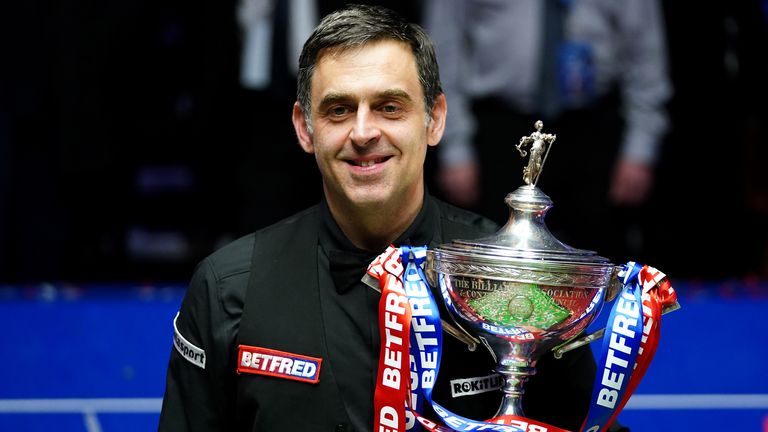This photograph captures a middle-aged man with a hint of gray in his dark hair, smiling as he holds a large silver trophy adorned with ribbons. He is dressed in a black tracksuit featuring a red and white "Betfred" logo, indicating a possible sponsorship. The trophy itself is topped with a statue of a human figure and decorated with red and blue ribbons that also bear the Betfred name in white text. The image is zoomed in on the man and his prize, rendering the background and other people blurry. The setting features a striking contrast between the dark, almost black upper background and the bright blue floor below, divided by a distinct white line. A partially visible individual in the distance, possibly a security officer, adds context to the otherwise celebratory focus of the photograph.